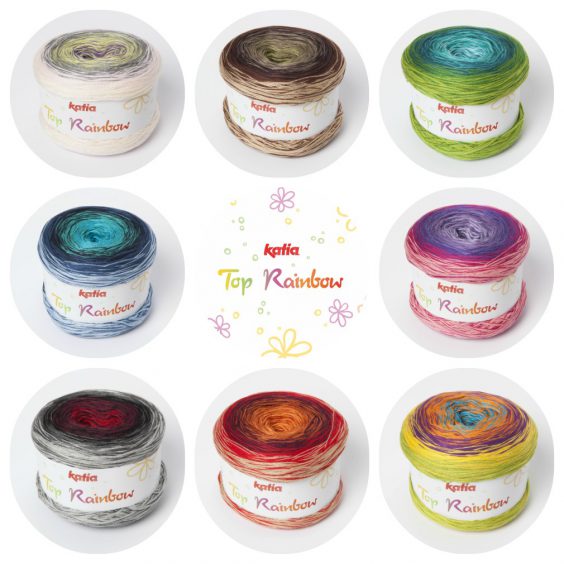The image features a carefully organized assortment of yarns in a grid layout, organized into three rows and three columns, totaling eight distinct skeins of yarn. The top row comprises three yarn balls: creamy beige on the left, brown in the middle, and green on the right. In the second row, the left yarn is blue while the right one is pink, with an empty middle space. The bottom row includes gray on the left, red in the center, and orange on the right. Each yarn skein is wrapped with a white label bearing the brand name "Katia Rainbow." The center of the pattern showcases the "Katia Rainbow" logo encircled by delicate flower designs in purple and yellow. The varied yarn colors span the spectrum, including shades of beige, light green, light blue, pink, orange, and yellow. This vibrant collection underscores the diverse color offerings of Katia Rainbow yarns, positioned neatly to emphasize the brand's commitment to high-quality and colorful options.